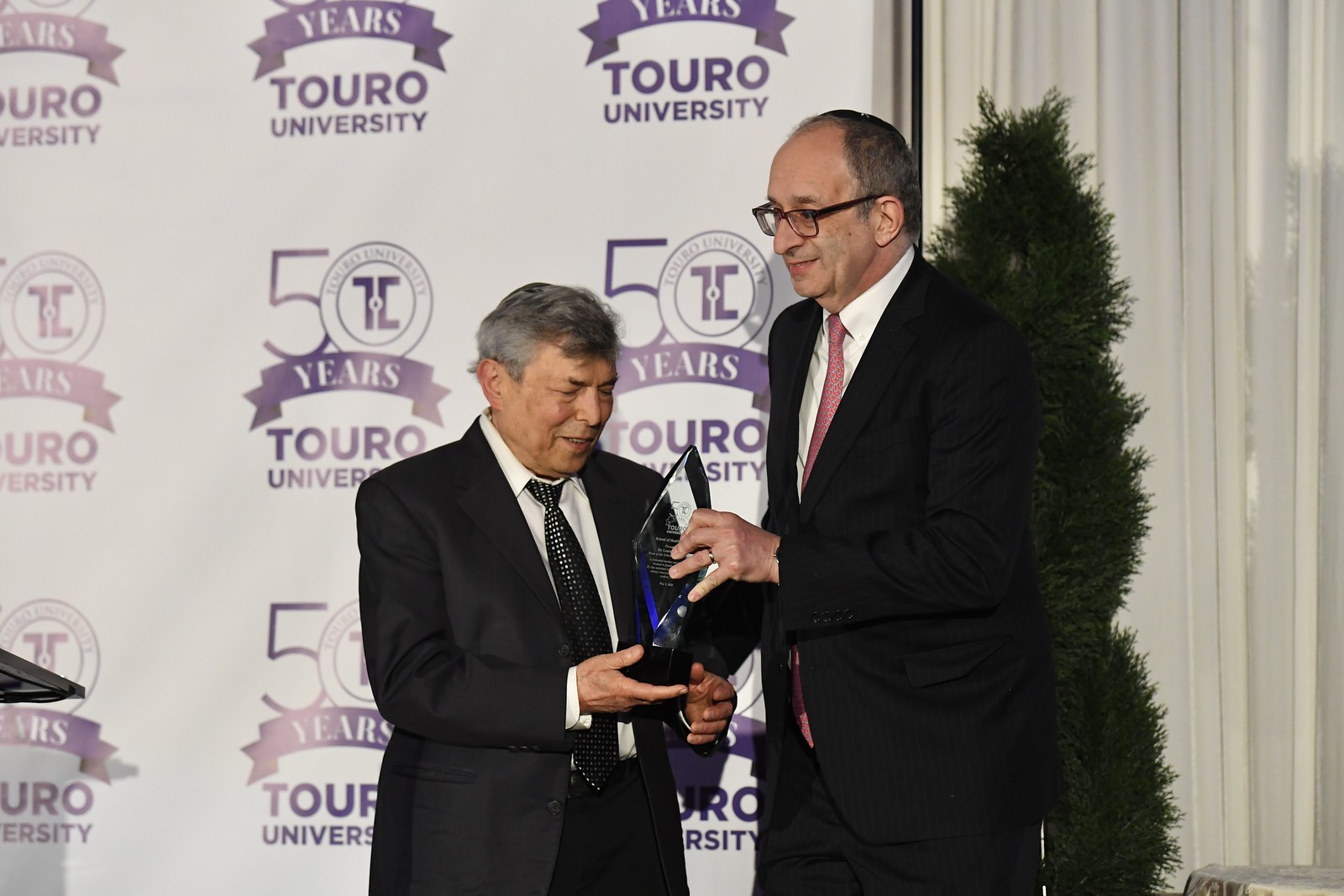This photograph captures an award ceremony at Touro University, commemorating its 50th anniversary. Dominating the left side of the image is a white backdrop adorned with purple "50 Years Touro University" logos, which repeats multiple times. On the right side, there are white plastic curtains creating a stage-like ambiance. A tall, dark green pine tree plant stands out behind one of the men. At the lower left, partially obscured, a black podium peeks into the frame.

In the center of the image, one man, significantly taller and balding, with glasses, is presenting a diamond-shaped glass award with a black base to another man. The taller man is dressed in a navy suit, white button-down shirt, and a pink tie. The recipient of the award, slightly shorter with gray hair, is wearing a dark gray suit paired with a silver and black tie and a white shirt. The scene exudes a formal and celebratory atmosphere, indicative of a special milestone for the university.